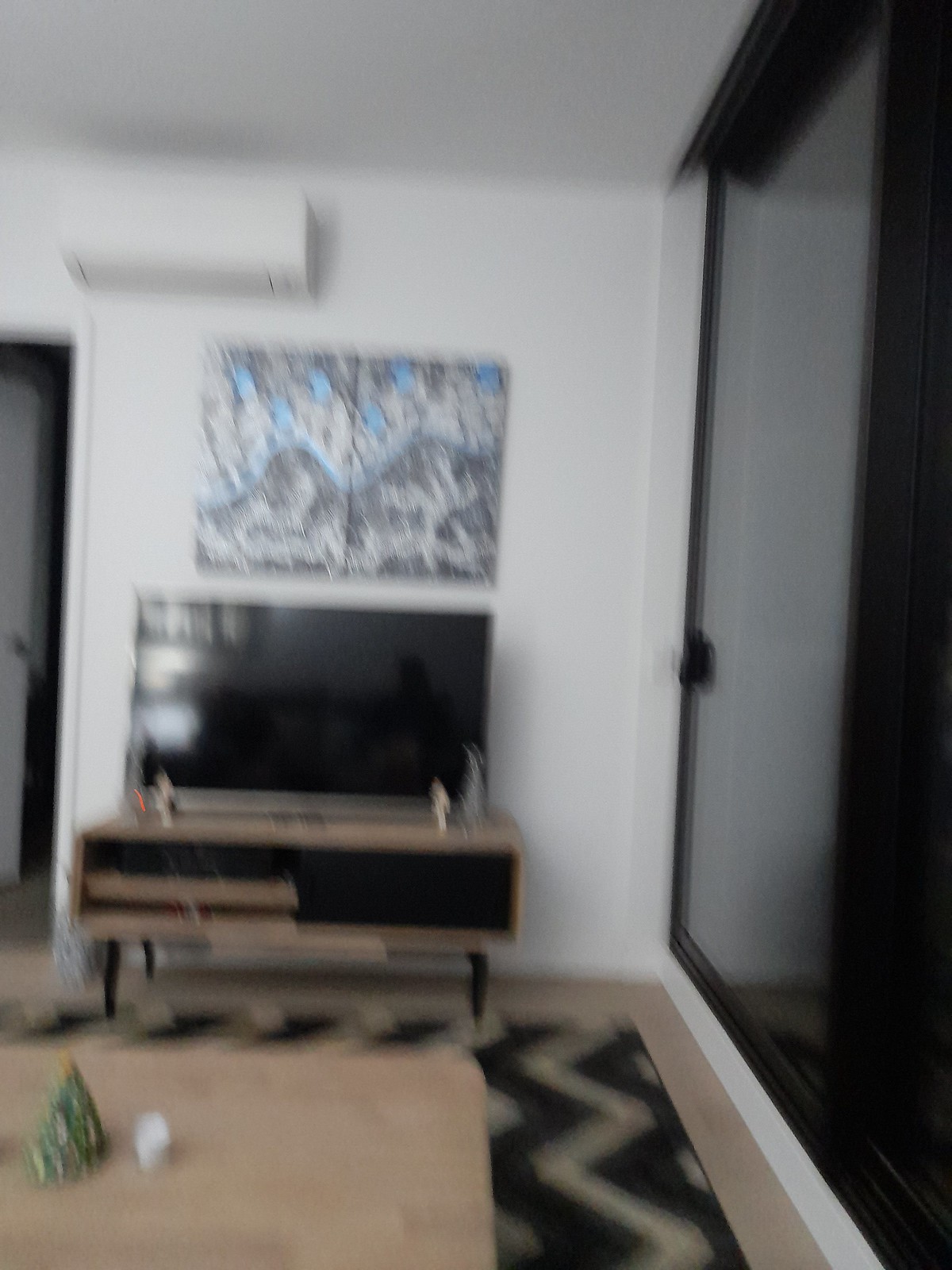This is a blurry image of a corner of a living room, depicting a cozy and detailed space. To the right, there is a large window or possibly a sliding glass door framed with black trim, giving a reflection due to the likely evening setting outside. Central to the room, a black screen television sits on a brown wooden TV stand, which is positioned against an off-white wall. Above the television hangs a distinctive picture, featuring black, white, and blue hues. Higher on the wall, an air conditioning or central AC unit is perceptible. To the left, a small portion of a doorway is visible. On the floor lies a brown area rug with a unique black border, adding texture to the room’s appearance. The overall dimensions and layout of the room suggest a comfortable living space, even though the image is out of focus.